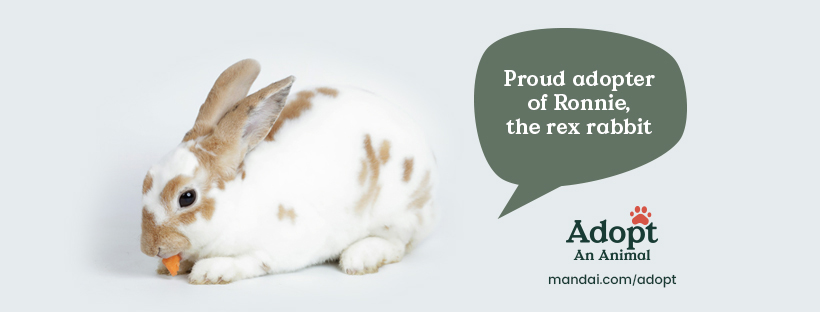This image serves as an advertisement for animal adoption, featuring a visually engaging design. The background transitions smoothly from white to a soft light green, creating a calming and inviting atmosphere. Positioned on the left-hand side of the image is a charming rabbit. The rabbit is primarily white with patches of tan and brown, happily munching on a bright orange carrot that protrudes from its mouth.

The rabbit is captured in a profile view, showcasing its left side. Its ears, adorned with black spots, stand tall and alert. While its fluffy tail and front paws are not visible, the rabbit’s content demeanor is evident as it enjoys its snack.

A speech bubble near the rabbit highlights text that reads, "Proud adopter of Ronnie the Rex Rabbit." The text is in white and is set against a dark sage green background, complementing the overall color scheme. Below, it encourages viewers to "Adopt an animal," with a red paw print playfully substituting the "P" in "Adopt." The URL "mandi.com/adopt" is displayed beneath this message, all in the same hunter green color as the speech bubble, guiding interested individuals on where to go for more information.